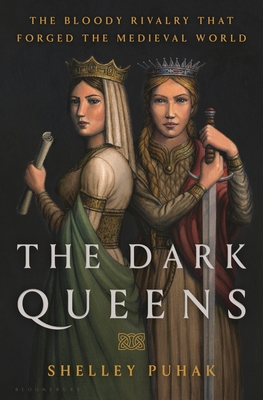The cover of the book "The Dark Queens" by Shelley Puhak features a dramatic, medieval-themed illustration set against a dark brown background. At the top, in orangey-yellow/gold text, it reads "The Bloody Rivalry That Forged the Medieval World." The title "The Dark Queens" is prominently displayed in large white letters in the bottom third of the cover, with the author's name, Shelley Puhak, in a matching yellow-orange/gold font at the bottom. Central to the cover are two painted women in medieval attire, both wearing crowns and facing the viewer. 

The woman on the left, adorned with a gold crown that features a veil at the back, has a regal appearance with her white dress and green cloak draped over her left arm. She holds a rolled-up scroll in her left hand and gazes towards us. The woman on the right, in a contrasting outfit of dark beige with a red sash, wears a silver tiara adorned with jewels. She holds a long sword, its blade resting on the floor though it is cropped out of the image. Both figures exude a sense of power and rivalry, emphasizing the book's historical and dramatic themes.